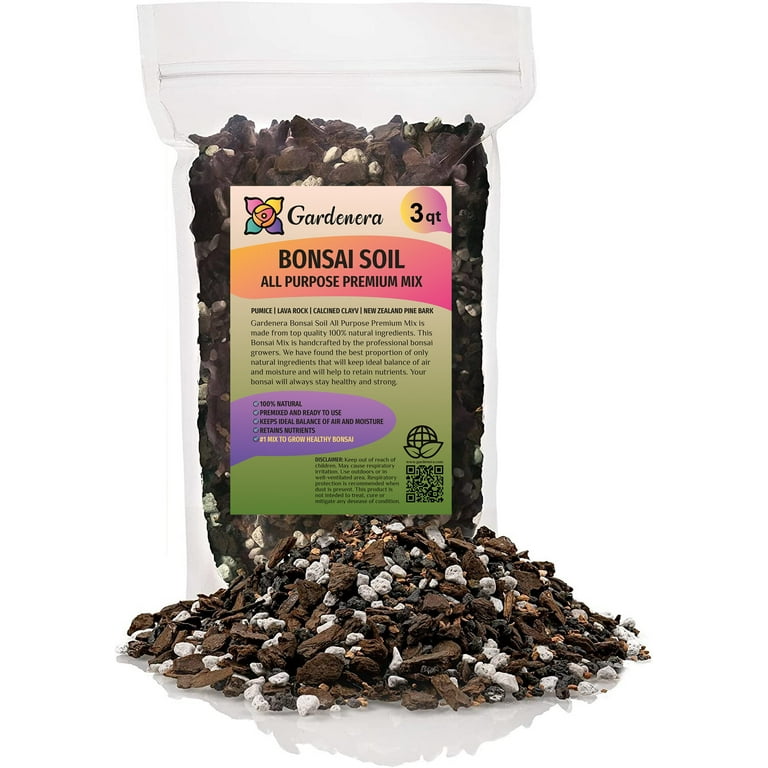The image depicts a clear zip-tied bag of Gardenera Bonsai Soil All-Purpose Premium Mix, prominently displayed with its label facing the camera. The label features a top white border with "GARDENERA" written in black letters and a colorful flower logo with pink, yellow, blue, and green petals and a red and yellow center. In the top right corner, a circle details "3 QT" indicating three quarts. An orange stripe below the white section announces "Bonsai Soil All Purpose Mix," and the remaining green area includes various instructions and a blue bubble near the bottom left with additional text.

In front of the bag lies a peaked pile of the soil, tapered towards the edges, composed of black, brown, and white rocks mixed with dirt, pebbles, and possibly twigs. The soil includes 100% natural, premixed components like pumice, lava rock, calcined clay, and New Zealand pine bark, making it ready to use for bonsai trees. The bag is slightly ripped at the bottom, allowing some of the mixed soil chunks to spill out. Additionally, a QR code on the front offers further information about the product.